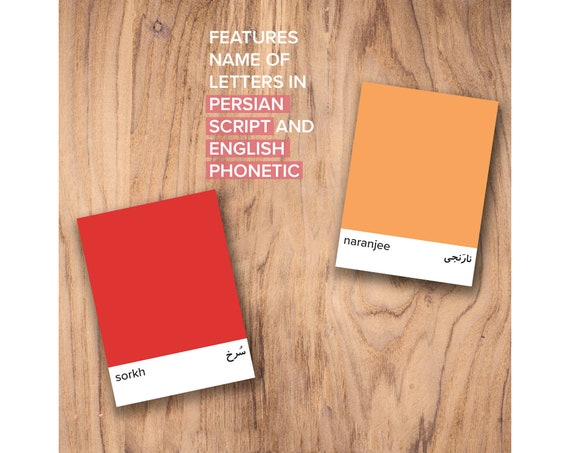The image appears to be an advertisement or product sample photograph. It features a wooden background with a medium brown, wavy wood grain pattern, giving it the appearance of a desk surface. The central text reads "Features names of letters in Persian script and English phonetic," with part of this text highlighted against a reddish background. 

To the right of the text, there are two color swatches resembling notepads or paint samples. The swatch on the left is a dark reddish color, while the one on the right is an orangish-brown. Both swatches have a white strip at the bottom featuring English phonetic spellings of Persian words. The left swatch reads "s-o-r-k-h" (Sorkh), and the right swatch reads "n-a-r-a-n-g-e-e" (Narangi). Each swatch also includes corresponding Persian script next to the phonetic spelling. The image overall conveys a clear and visual representation of how Persian letters and their English phonetic equivalents are featured.